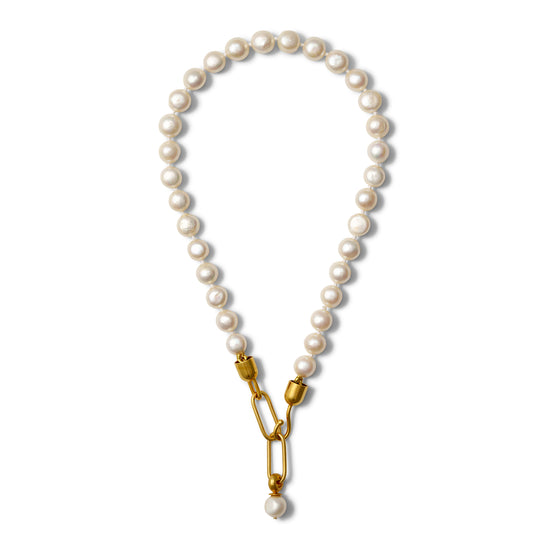The image showcases a pearl necklace set against a pure white background. The necklace is composed of approximately 20 to 30 rounded, shiny pearl beads that appear to be tightly strung together, creating a luminous effect as the light reflects off them. The pearls have a smooth, polished surface, suggesting they might be made of plastic. At one end of the necklace, there is a sturdy golden or bronze hook clasp, which fits seamlessly into two small bronze loops at the opposite end. These two ends meet at a final single white pearl, completing the elegant and compact design of the necklace. The overall length suggests it's just sufficient to encircle the neck, emphasizing its use as a piece of refined jewelry.